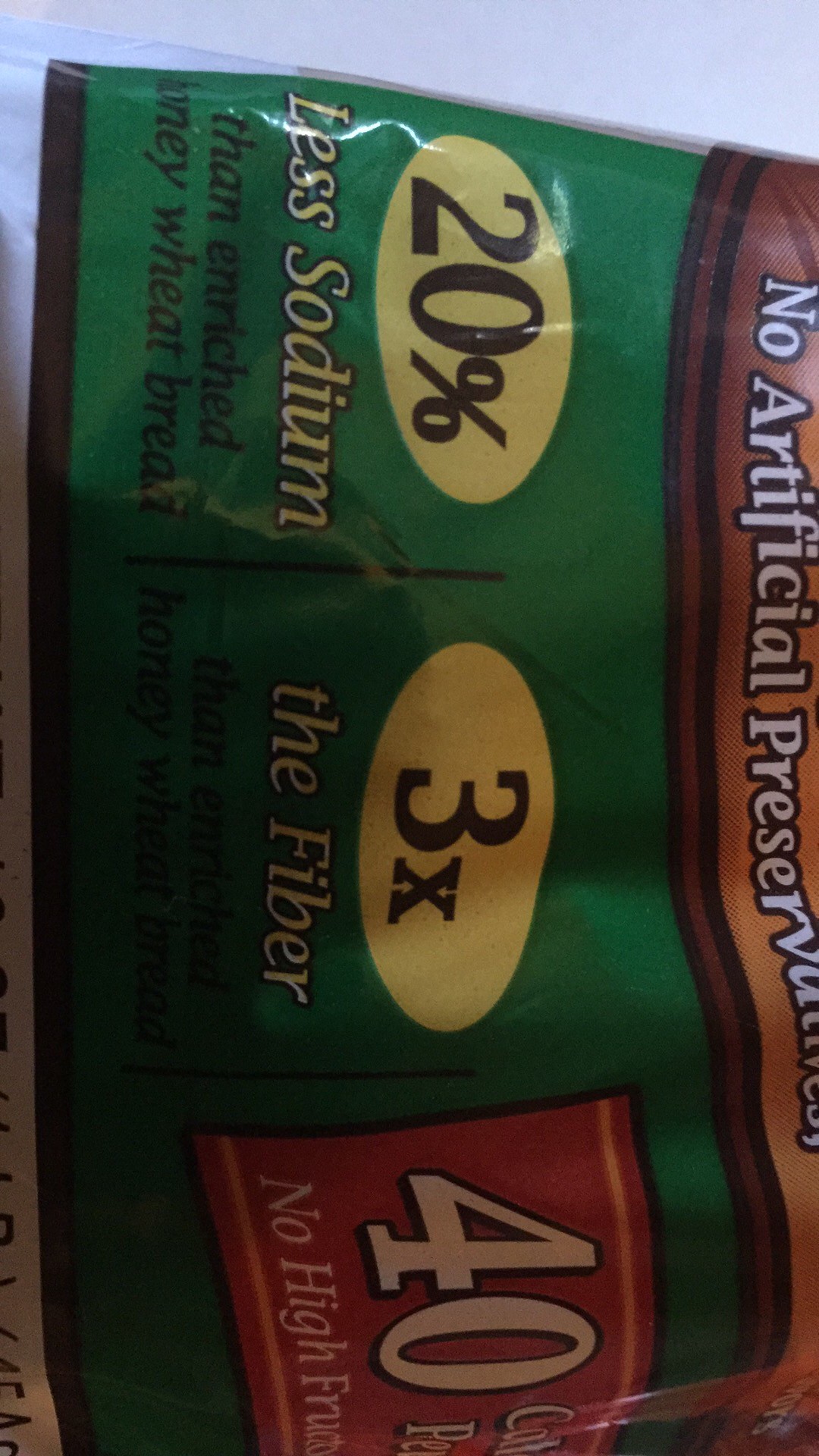The image showcases the side view of a food product's front packaging, requiring a tilted head to read the text properly. Prominently displayed at the top, "No Artificial Preservatives" is clearly visible. The packaging features three distinct nutritional labels: one indicating "20% Less Sodium than Enriched Honey Wheat Bread," another highlighting "Three Times the Fiber," and the last one suggesting "40 Calories per Piece," though the exact number of calories is partially obscured. The text also mentions the absence of high fructose corn syrup. The packaging boasts a predominantly green color scheme, accented with shades of brown, yellow, and a touch of red.